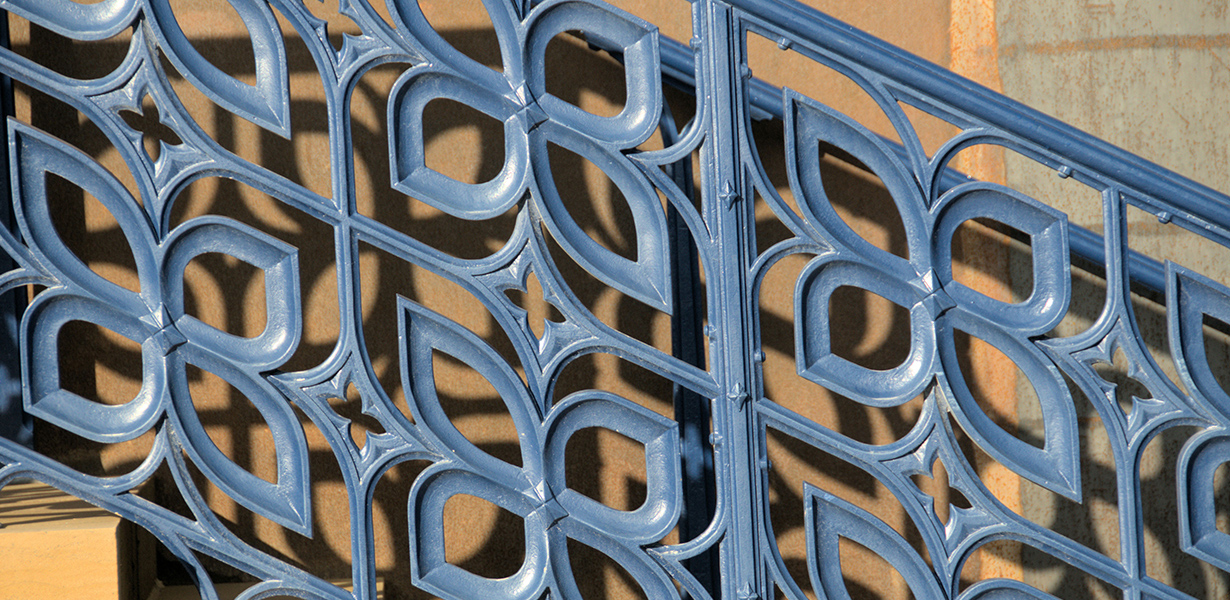This rectangular image, approximately twice as wide as it is tall, captures a close-up view of an ornate guardrail ascending a set of stairs, emphasizing its intricate design. The focal point is the railing, painted a grayish-blue tone, featuring a repeating pattern of four intersecting leaves forming an X-shape, with smaller, diamond-like details at the intersections. This decorative railing runs diagonally from the bottom right to the top left. In the lower left corner, a light brown step is just visible, possibly wooden or a similarly colored concrete. The background reveals a partially gray and brown concrete wall, with a subtle black shadow behind the railing, highlighting its delicate yet possibly sturdy structure, though the image leaves it somewhat ambiguous.